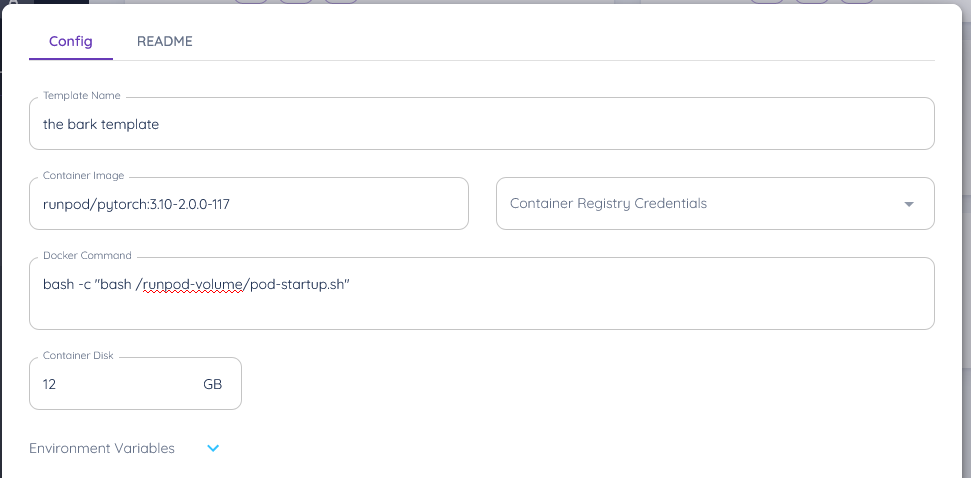This image depicts a cropped screenshot of an admin configuration panel for website IT, set against a clean white background. At the top, in bold blue letters, the word "CONFIG" is prominently displayed and emphasized with a blue underline. Just to the right, "READ ME" is written in all caps, bold, and gray.

Underneath, there is a notably extensive text box labeled "Template Name", with the words "the bark template" typed inside in lowercase letters. This section is followed by a larger box on the left marked "Container Image", which contains a link: "run pod/PyTorch.3.10-2.0.0-117".

To the right of this, a dropdown menu is visible displaying the selected option "Container Registry Credentials". Below this section, another large text box is titled "Docker Command", within which a specified command is visible. Further down the interface, the label "Container Disk" indicates a setting configured to 12 gigabytes, positioned at the bottom left. Lastly, at the very bottom, the term "Environment Variables" is present alongside a dropdown menu, though the remaining content is cropped out from the screenshot.